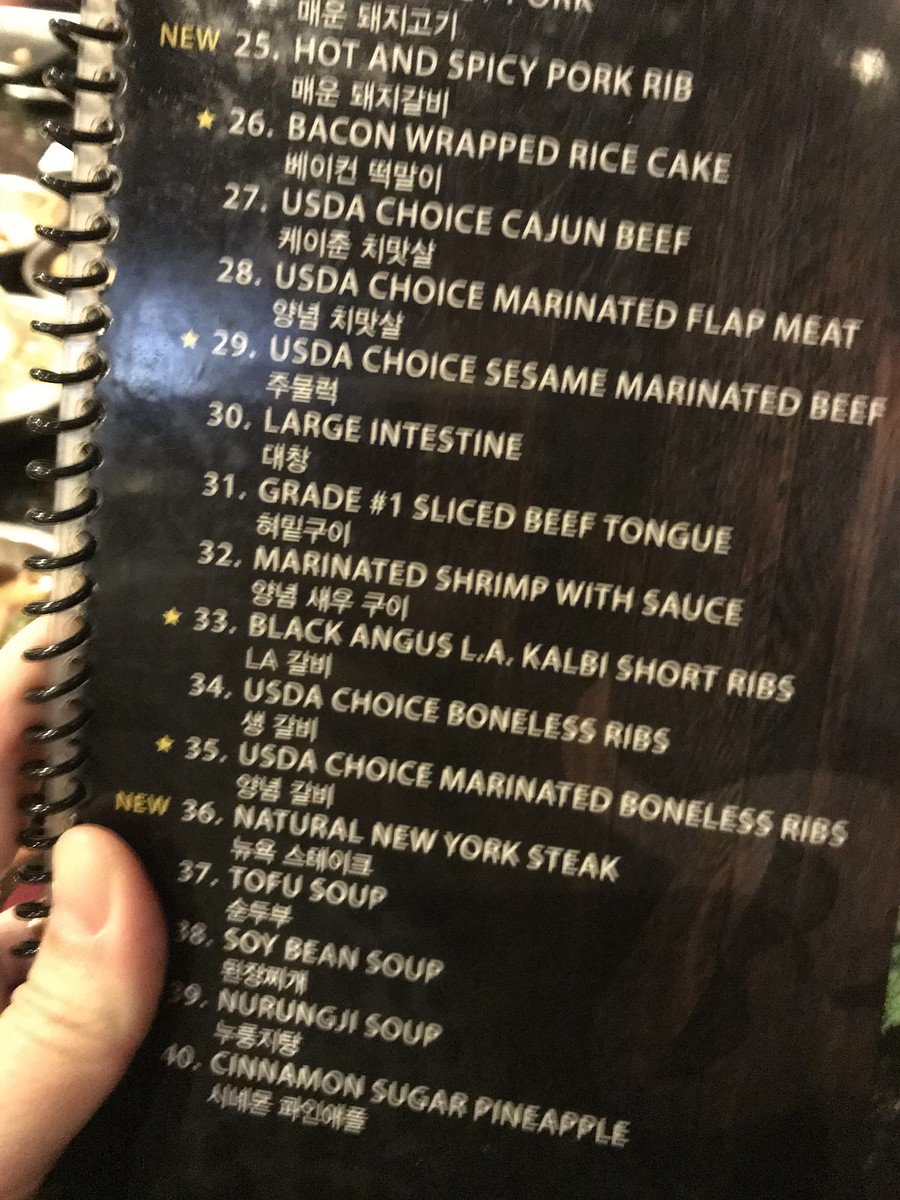The image showcases a page from a spiral-bound menu, featuring newly introduced dishes. The page, held up by a person's hand, displays their thumb in the front and fingers behind, against a backdrop of food on a counter. You can see several white plates with food to the left of the menu. The spiral binding is black, and the page prominently features the word "NEW" accompanied by Asian characters. This particular menu page lists items starting from number 25, suggesting continuation from the previous page. The dishes include:

1. Hot and Spicy Pork Rib
2. Bacon Wrapped Rice Cake
3. USDA Choice Cajun Beef
4. USDA Choice Marinated Flat Meat
5. USDA Choice Sesame Marinated Beef
6. Large Intestine
7. Grade No.1 Sliced Beef Tongue
8. Marinated Shrimp with Sauce
9. Black Angus Kalbi Short Ribs
10. USDA Choice Boneless Ribs
11. USDA Choice Marinated Boneless Ribs
12. Natural New York Steak
13. Tofu Soup
14. Soybean Soup
15. New Ranch Soup
16. Cinnamon Sugar Pineapple

The detailed caption captures the essence of the image, indicating the novelty and variety of the dishes presented.